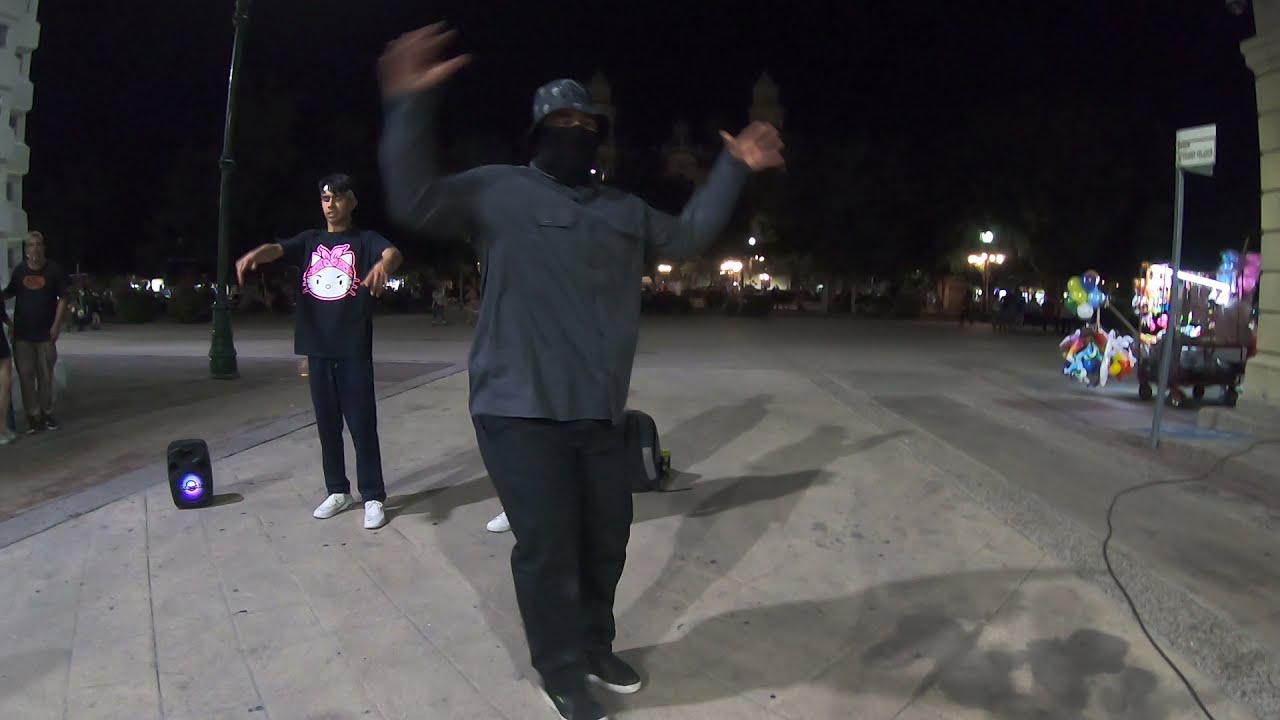In this somewhat blurry, horizontally aligned nighttime photo, the black sky forms the upper background, contrasting against tall buildings and a street scene below. The main focus is two men in the foreground seemingly engaged in a dance or street performance. The man at the front is dressed in black pants, black shoes with white soles, and a dark gray long-sleeve button-down shirt. He wears a black COVID mask and a gray and white bucket-style hat, with his arms raised mid-motion, which appear somewhat blurred. 

Behind him, slightly to the left, another man in a black outfit catches attention. This second man wears a black shirt featuring a Hello Kitty graphic, black pants, and white shoes, with his arms extended in a zombie-like stance and eyes closed. At his feet is a boombox illuminated with blue, pink, and green lights. 

In the background to the left, another man in a black t-shirt and brown pants stands idly. On the right side, a blurred street sign mounted on a pole is visible, alongside some balloons on the ground. There is also a small figure—possibly a woman or child—near the balloons, adding more life to the nighttime urban tableau. The scene appears to take place in the middle of a road or walkway.